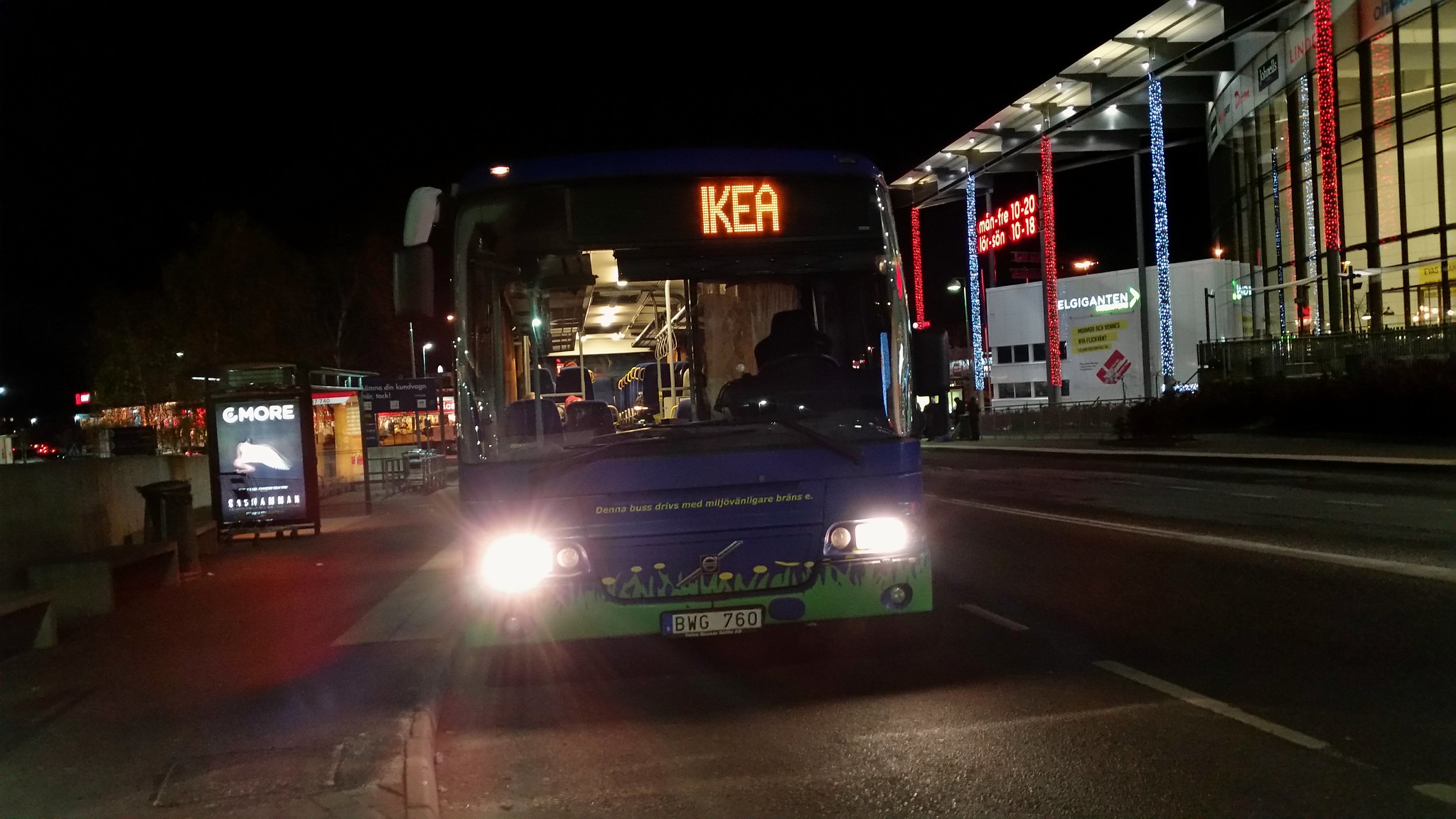In this nighttime photograph, we see a front view of a public transportation bus with its headlights on. The destination sign at the top, lit up in orange and red letters, displays "IKEA." The bus itself has a dark blue upper section with a lime green trim around the bottom. The license plate reads BWG 760, and the side of the bus features the text "Dana Bus Drive Mid-Melkvillain Brain."

In the urban background, there are illuminated signs on the far left, displaying various advertisements, and on the far right, a brightly lit building which could be a convention center or sports stadium. The building has a sign indicating its open days and times. Adjacent to this structure, visible through a large window and glass doors, is a brightly lit lobby. Further left in the scene, another building, possibly an office, is partially visible. The bus appears to be stationary, likely at a bus stop, in a semi-empty city street.